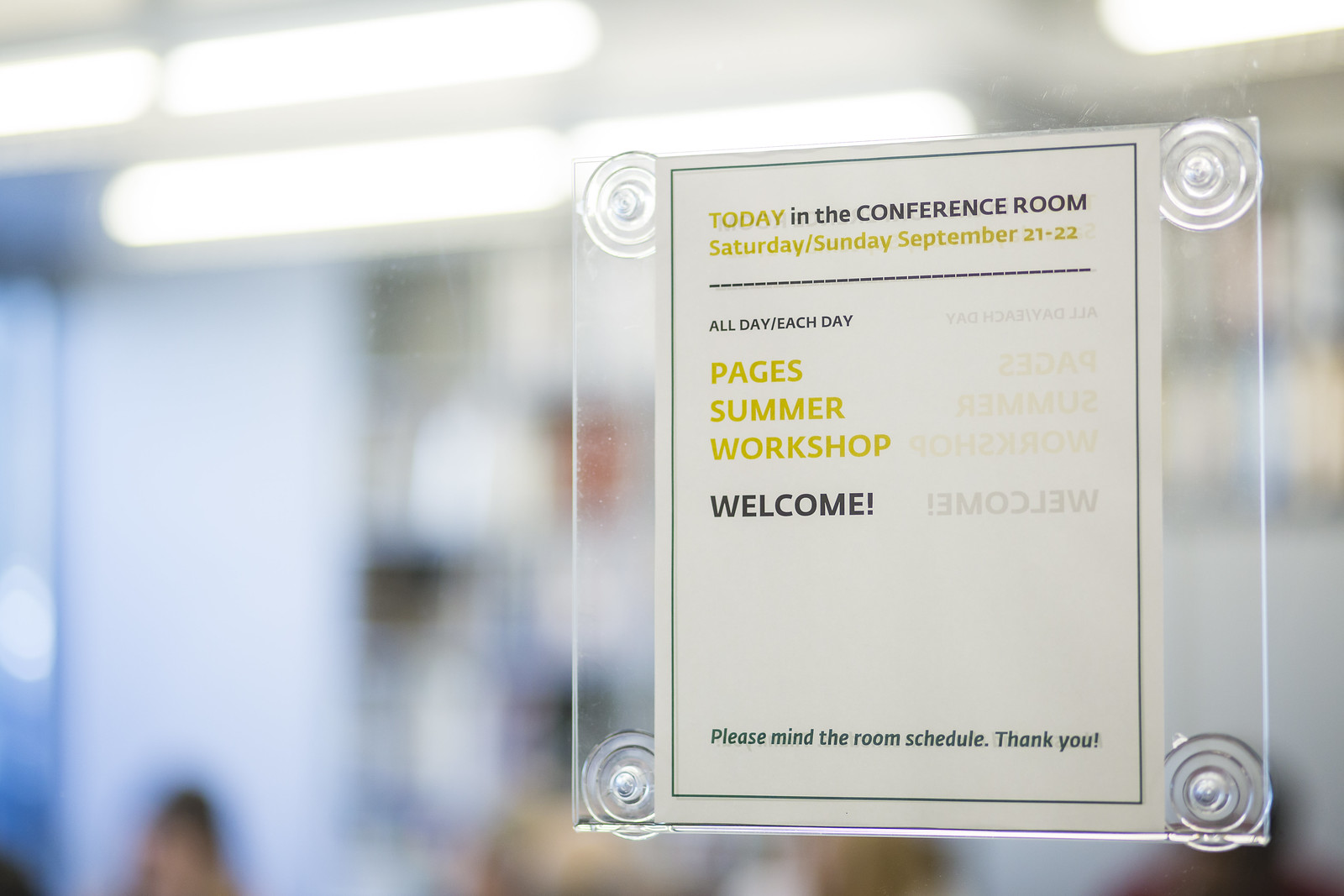The photograph captures a sign affixed to a glass wall, likely a door, using small suction cups. The main focus of the image is the white sheet of paper with multi-colored text in yellow, black, green, and gray. The text reads, "Today in the conference room, Saturday/Sunday, September 21-22. All day each day. Stages Summer Workshop. Welcome. Please mind the room schedule. Thank you." Behind the glass wall, you can make out blurry figures of people in what appears to be an office setup with a white wall displaying a painting. The background is illuminated with ceiling lights, indicating the presence of activity within the room.